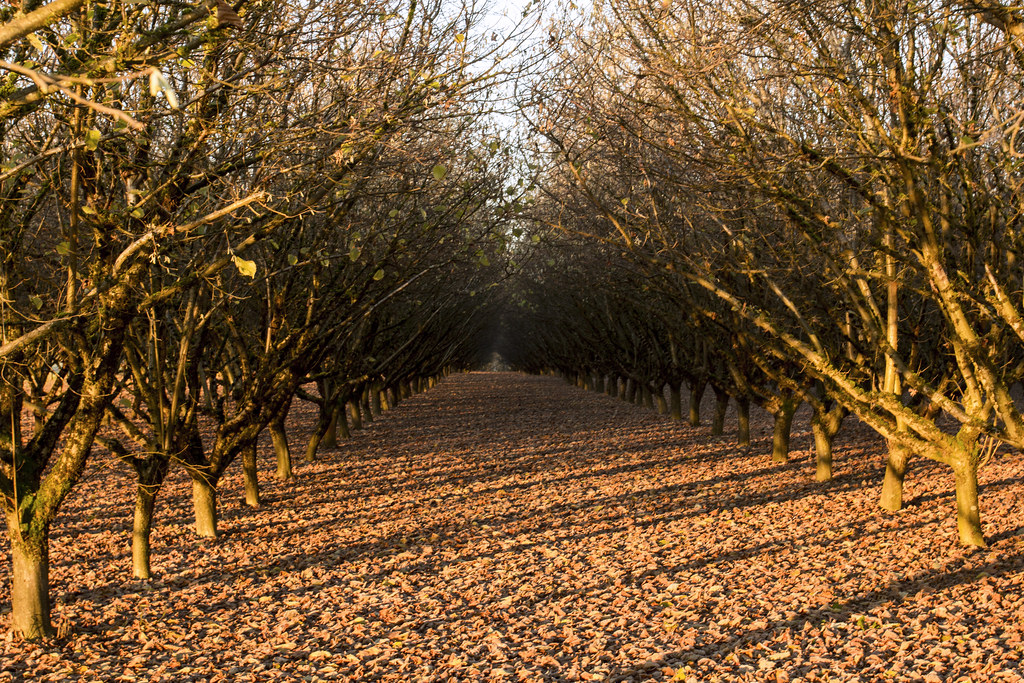The photograph showcases a serene avenue of an orchard with rows of barren trees, possibly apple, pear, orange, or lemon trees, creating a naturally arched pathway. The trees are aligned in neat, straight lines flanking a central dirt path. The ground is covered in a tan, dark brown material that appears to be decomposing leaves, reflecting the end of the harvest season or wintertime. The trees are mostly devoid of leaves, with just a few sparse remnants clinging to the branches. The avenue culminates in a distant wooded area, where the leafless branches form a delicate lattice against the faintly visible sky.